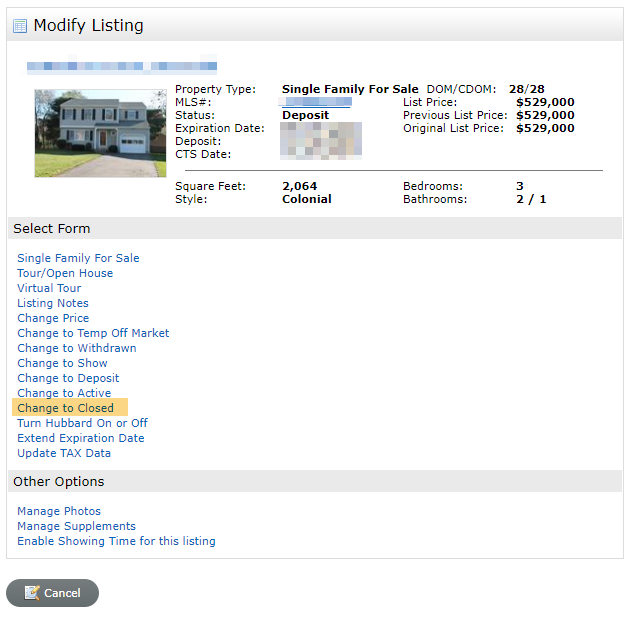**Detailed Caption:**

The image depicts an online portal, likely from a real estate website, showcasing a substantial suburban home modernly styled in the Colonial architectural tradition. The listing, marked as a single-family property for sale, reveals key details though some information is obscured. The property status is tagged as 'deposit', with sections for expiration date, deposit, and CTS date displayed but grayed out. This home, listed at $529,000 (consistent with its previous and original list price), offers 2,064 square feet of living space. The residence comprises three bedrooms, two full bathrooms, and one half-bathroom.

Further down, the interface presents numerous interactive options: select form, initiate a virtual tour, schedule an open house, input listing notes, adjust the listing price, or modify the market status to 'temporarily off market' or 'withdrawn'. At the moment, the option to 'change to closed' is prominently highlighted, suggesting that the user might be in the process of finalizing the listing status. Additional functionalities allow the user to turn features on or off, extend the expiration date, update tax data, manage property photos, add supplements, and enable showing times for this listing. The interface clearly serves as a comprehensive tool for realtors to manage property listings efficiently.